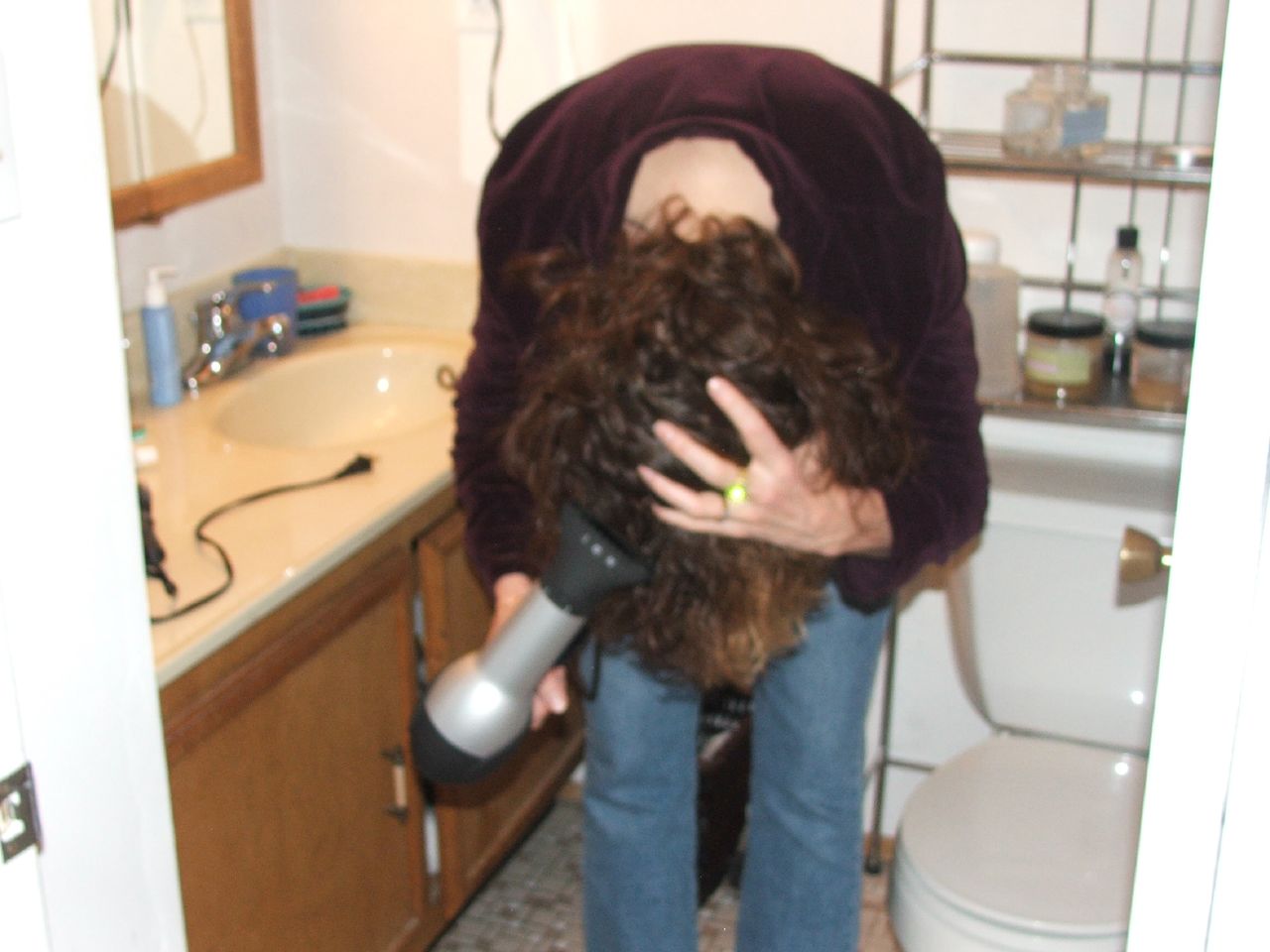The photo captures a woman, whose gender might not be immediately obvious, positioned in a pristine bathroom. She is bent over, blow-drying her wavy, reddish-brown hair with a silver hairdryer equipped with a black diffuser, her head tipped down so only the top is visible. She wears a burgundy long-sleeve shirt and blue jeans, with a shiny, greenish-yellow ring on her middle finger of her left hand, which is used to fluff her hair. Her right hand holds the hairdryer close to her hair, which is already mostly dry.

The bathroom is notably clean and organized. The woman stands between a beige porcelain sink with brown wooden cabinets beneath it and a white toilet. Above the toilet is a silver shelving unit holding various bathroom products and possibly a Kleenex box. The sink area is cluttered modestly with a soap bottle, a cup, and a curling iron. There is a visible wall-mounted mirror with a brown wood trim behind the sink. The bathroom floor appears to be brown tile, although specifics of the flooring are not very clear.

The entire scene conveys a sense of the woman getting ready for her day, meticulously using her hairdryer in the small, well-kept bathroom space.